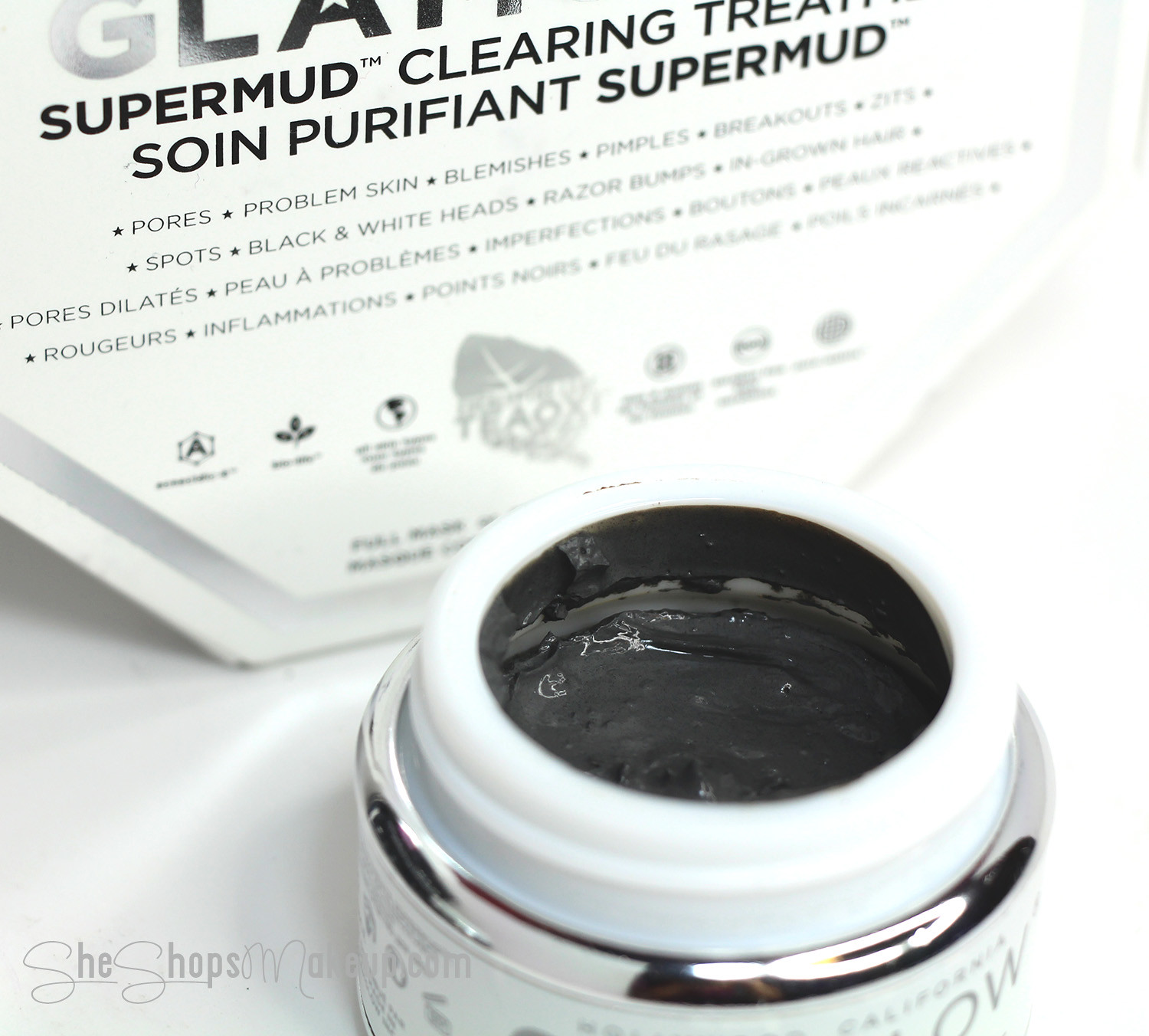The photograph features a black and white themed product prominently displayed in the forefront. This product is a jar of "Super Mud Clearing Treatment," an intensive skincare solution designed to address various skin issues such as pores, problem skin, blemishes, pimples, blackheads, whiteheads, breakouts, razor bumps, and ingrown hairs. The jar is open, revealing its contents: a black gooey substance functioning as the mud mask. Surrounding the product, there are several small symbols indicating its environmentally safe and all-natural benefits. Notably, the text on the product includes both English and what appears to be French translations, with phrases like "Soin Purifiant" following the English descriptors. The background of the image includes watermarks and additional text that is partially obscured, but hints at being related to eco-friendly and consumer safety assurances.